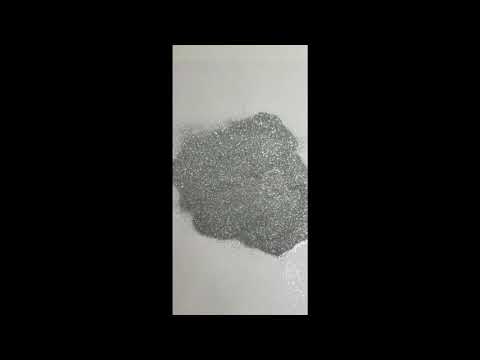The image depicts a central mass that resembles a face in shape but is made up of intricate lines, curves, and circular patterns, evoking the look of a topographical map or brain-like material. This mass is a darker gray and sits on a light gray or white background, occupying almost the entire width of the inner rectangular space. The inner space is surrounded by a prominent black border. The central mass appears granular and irregular, with some portions, especially on the top left, smeared into the background, giving it a grainy, slightly shiny texture that reflects light. This central feature looks almost like silver glitter or metallic dust piled up in a somewhat circular shape, situated in the middle of what might be a piece of paper or waxed paper. The overall resolution of the image isn't very high, making the granular details appear with varied light reflectivity.